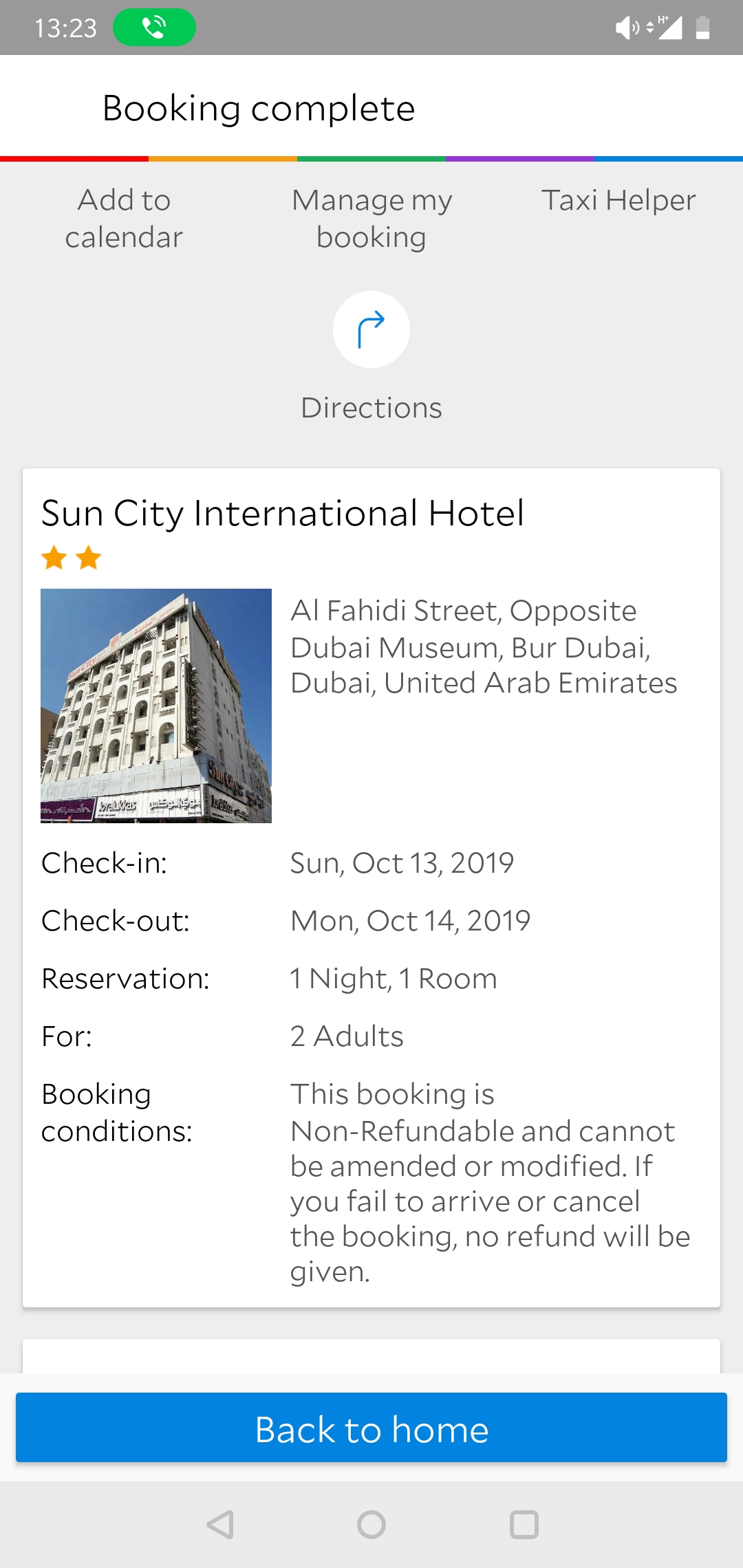The top of the image features a long horizontal gray bar displaying the time "13:23" on the left side. To the right of the time, there is a green circle with an icon of a white phone inside it. Further to the right, a vertically placed battery icon shows a very low battery level, indicated by a small white segment.

Below this bar, the text "Booking Complete" is prominently displayed and underlined by a multi-colored horizontal line that transitions from red to orange, green, purple, and blue. Under the red section of this line is the text "Add to Calendar," followed by "Manage My Booking," and "Taxi Helper."

Beneath this section, there is a white circle with a blue arrow pointing to the right and the word "Directions." 

The next section contains the text "Sun City International Hotel" with two orange stars below it, accompanied by an image of a white building with approximately five floors. The address provided is: "Al-Fahidi Street, opposite Dubai Museum, Burj Dubai, United Arab Emirates."

Following this, the check-in date is listed as "Sunday, October 13th, 2019," and the check-out date as "Monday, October 14th, 2019." The reservation details specify "One night, one room for two adults." The booking conditions note that "This booking is non-refundable and cannot be amended or modified."

At the bottom of the image, a long blue bar contains the text "Back to Home."